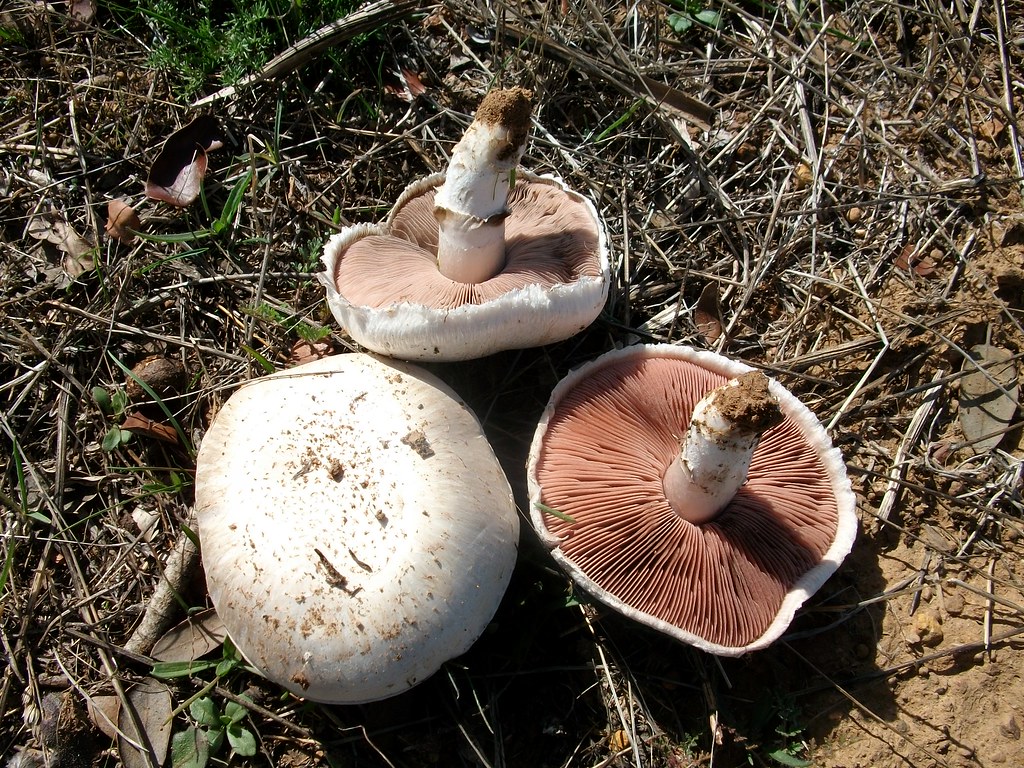In this detailed outdoor photograph taken during the daytime, the focus is on three mushrooms laying on a patch of dirt mixed with brown, twiggy debris, sparse green grass, and dead leaves. The largest mushroom, situated in the lower-left section of the image, displays its white top adorned with black speckles. To its right lies another mushroom, showing its underside with a white stem and a light brown gill structure comprising several linear strands. Above these, a third mushroom also reveals its underside, similar in coloration with a white stem and a lighter brown gill network. All mushrooms appear freshly displaced, as evidenced by the dirt clinging to their stems and caps. Various shades of brown leaves and small patches of green growth are scattered throughout the background, enhancing the natural setting. Close to the lower-center of the image, a slightly pointed oval leaf with a visible stem is partially obscured by sticks, adding to the scene's intricate detail.